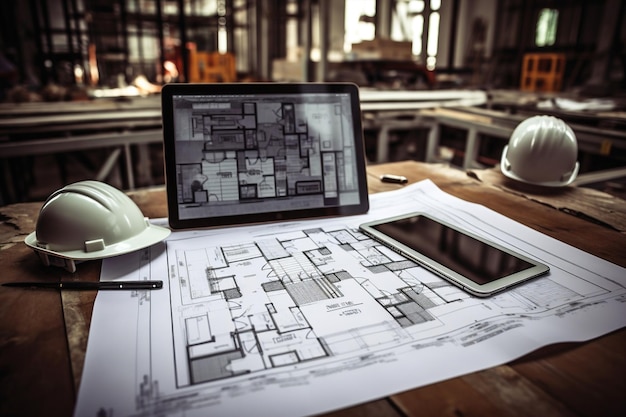This detailed photograph depicts a well-organized workstation set up on a U-shaped desk, showcasing one of its segments made of worn brown wooden planks, giving it a rustic feel. At the center of the desk is an upright iPad, accompanied by a cell phone and a white hard hat, which rests on top of a white sheet resembling a building blueprint. A pen is also placed on the blueprint, indicating ongoing work. Nearby, an additional hard hat is positioned just a few inches away on the table. The background reveals a room under construction, with visible vertical and horizontal beams allowing light to filter through. Various construction-related objects scattered around emphasize the active site environment.